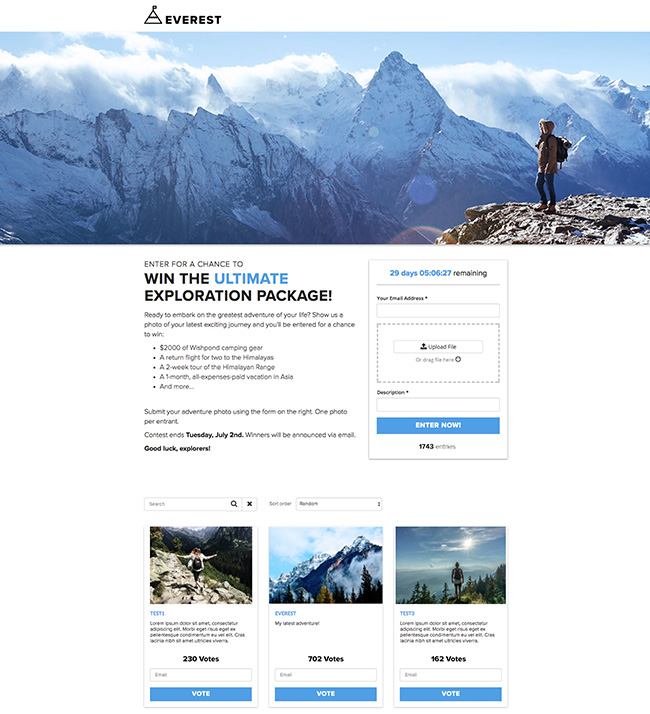**Caption:**

At the pinnacle of exploration, under the bold title "Everest," a lone adventurer stands at the brink of a cliff, gazing out at the majestic, snow-covered peaks of the Himalayas. The figure, cloaked in a heavy wool coat with a hoodie, complete with an array of professional hiking gear strapped into their bulky backpack, epitomizes the spirit of the ultimate explorer. The scene is awe-inspiring and grand, a breathtaking panorama that captures the essence of adventure and the allure of untouched nature.

Beneath this evocative image, an enticing challenge beckons: "Enter for a chance to win the ultimate exploration package." The call to action stirs the soul with promises of unparalleled adventure. "Ready to embark on the greatest adventure of your life?" it asks. Participants are prompted to share a photo of their latest thrilling journey for a chance to win an extraordinary prize package. The rewards include $2,000 worth of Wish Pond camping gear, a return flight for two to the Himalayas, a two-week tour of the Himalayan range, a one-month all-expenses-paid vacation in Asia, and more.

A countdown clock, prominently displayed on the right, shows 29 days and 5 hours remaining until the contest ends on Tuesday, July 2nd. Entrants can submit their adventure photo via a form on the right, allowing for one photo per entrant. Below, an email address field and a photo upload section make participation easy. Additional pictures showcasing the stunning beauty of various locations in the Himalayas further fuel the wanderlust of potential contestants.